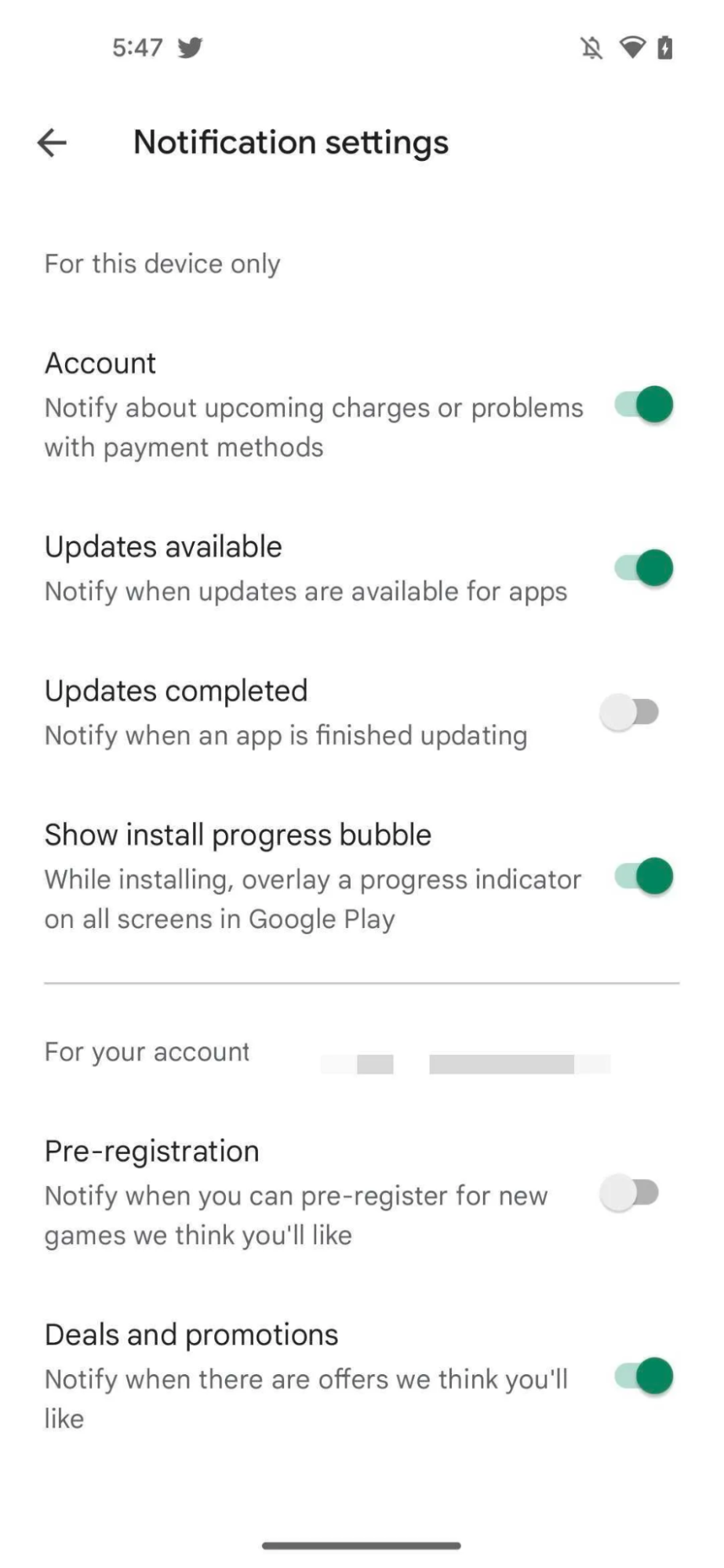The image depicts the notification settings interface on a smartphone with a white background and black text. At the top, it prominently displays "Notification Settings." On the left side, a section labeled "For this device only" is visible, indicating settings that apply solely to the device.

1. **Notification about upcoming charges and payment method issues**: This setting is active, with its toggle switch positioned to the right and displayed in green.
   
2. **Updates available**: This option is also enabled, with its corresponding toggle switch to the right and green, indicating notifications will be sent when updates for apps are available.

3. **Updates completed**: This setting is disabled, showing a grey toggle switch pushed to the left, meaning notifications for completed app updates will not be received.

4. **Show installed progress bubble**: Enabled, this setting will show an overlay progress indicator during app installations across all screens in Google Play, as indicated by the right-positioned green toggle switch.

Below the device-specific settings, a section titled "For your account" appears, with the account details obscured in grey.

1. **Pre-registration**: This notification, indicating when you can pre-register for new games, is turned off, with its grey toggle switch set to the left.

2. **Deals and promotions**: This setting is active, signaled by a green toggle switch to the right, allowing notifications for offers and promotions believed to be of interest.

This detailed configuration enables the user to manage various types of notifications related to app updates, financial activity, and promotional content effectively.